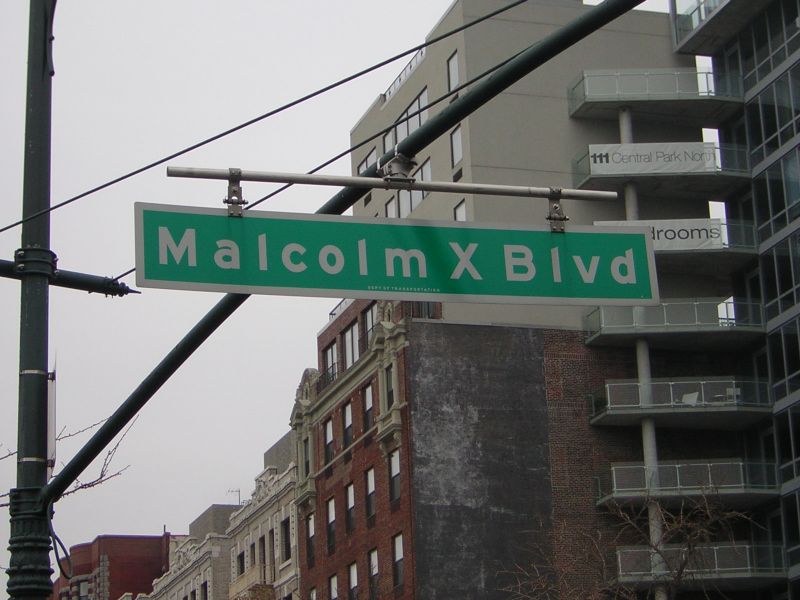The photograph captures an urban scene, evidently set in America, marked by a distinctive green street sign with white lettering that reads "Malcolm X BLVD." This sign hangs from an aluminum bar attached to a street pole that also supports a streetlight and various telegraph wires crossing above. The image is taken from an outdoor, street-level perspective, showcasing a row of multi-storied, brick and white apartment buildings extending diagonally from the lower left to the upper right of the frame. These buildings are reminiscent of New York's architectural style, characterized by repetitive glass windows and ornate detailing along the rooftops. To the far right, a high-rise building features several balconies, one of which prominently displays a banner reading "Central Park North." The far left of the image includes another streetlight, with telegraph wires stretching diagonally above. The sky appears gray and overcast, adding to the urban atmosphere. There are no people, animals, plants, flowers, trees, or vehicles in sight, emphasizing a quiet moment in the bustling city environment.